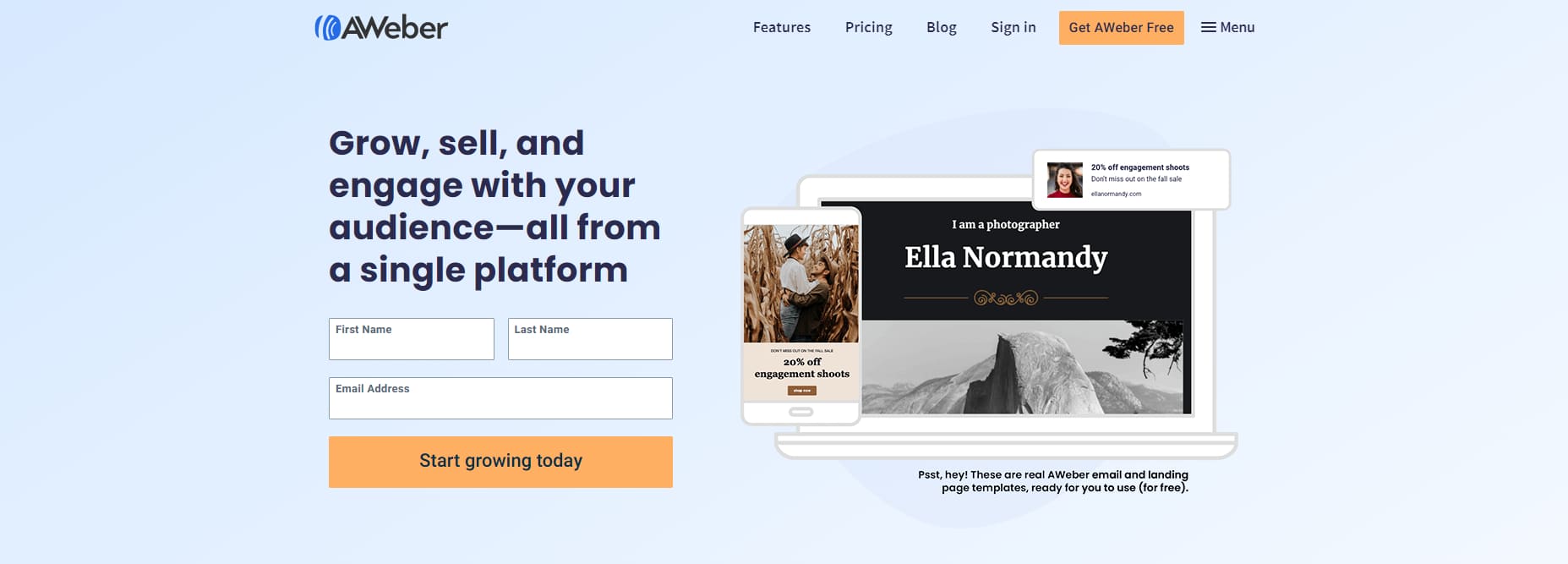The background of the scene is a soothing powder blue, giving it a calm and inviting appearance. At the top, in bold black letters, it reads "A-W-E-B-R." Beneath this, also in black text, is the tagline: "Grow, sell, and engage with your audience from a single platform." 

The central part of the image features two white boxes outlined with black borders. The first box is labeled "First Name" and the second one is labeled "Last Name." Adjacent to these is a longer box that spans their combined width, designated for entering an "Email Address." An orange box with black text encourages action with the words "Start Growing Today."

At the very top of the image, several navigation tabs are displayed in black, including "Features," "Pricing," "Blog," and "Sign In." An additional orange rectangle stands out with the call-to-action "Get AWeber Free." 

On the right side, there is an icon consisting of three black lines, typically representing a menu.

A prominent image of an animated white laptop and phone set against a black background catches the eye. On the screen of the laptop, it declares in black text, "I am a photographer, Eleanormity." Below this, it continues, "These are real Weber email and landing page templates ready for you to use for free."

The animated phone screen displays an image of two people hugging in a cornfield, along with the text "20% off engagement shoots" in black. 

The entire composition is meticulously organized, creating a cohesive and visually appealing layout.